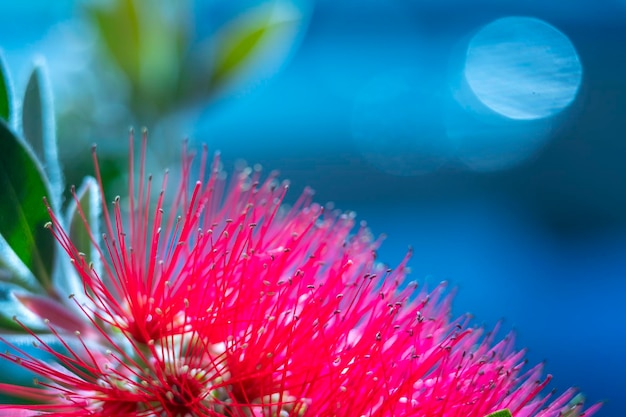In this detailed macro photograph, the focus is on the bright pink stamens of a flower, potentially a spider lily or a bottle brush plant, characterized by red, spiky, brush-like filaments with small, dark black or brown tips. These delicate fibers extend outwards, resembling fine needles or hair-like structures. Surrounding the stamens on the left side, there are some green, narrow leaves, with the sharper leaves contrasted against a blurred background, hinting at frond-like structures. The background is predominantly a gradient of blues, varying from lighter to darker hues, interspersed with small white circles indicating lens flare or light reflections. In the upper left, a reflected moon-like glow adds to the ethereal quality of the scene. The overall composition suggests an underwater or outdoor environment during the daytime, with the main subject in sharp detail against a beautifully blurred backdrop.